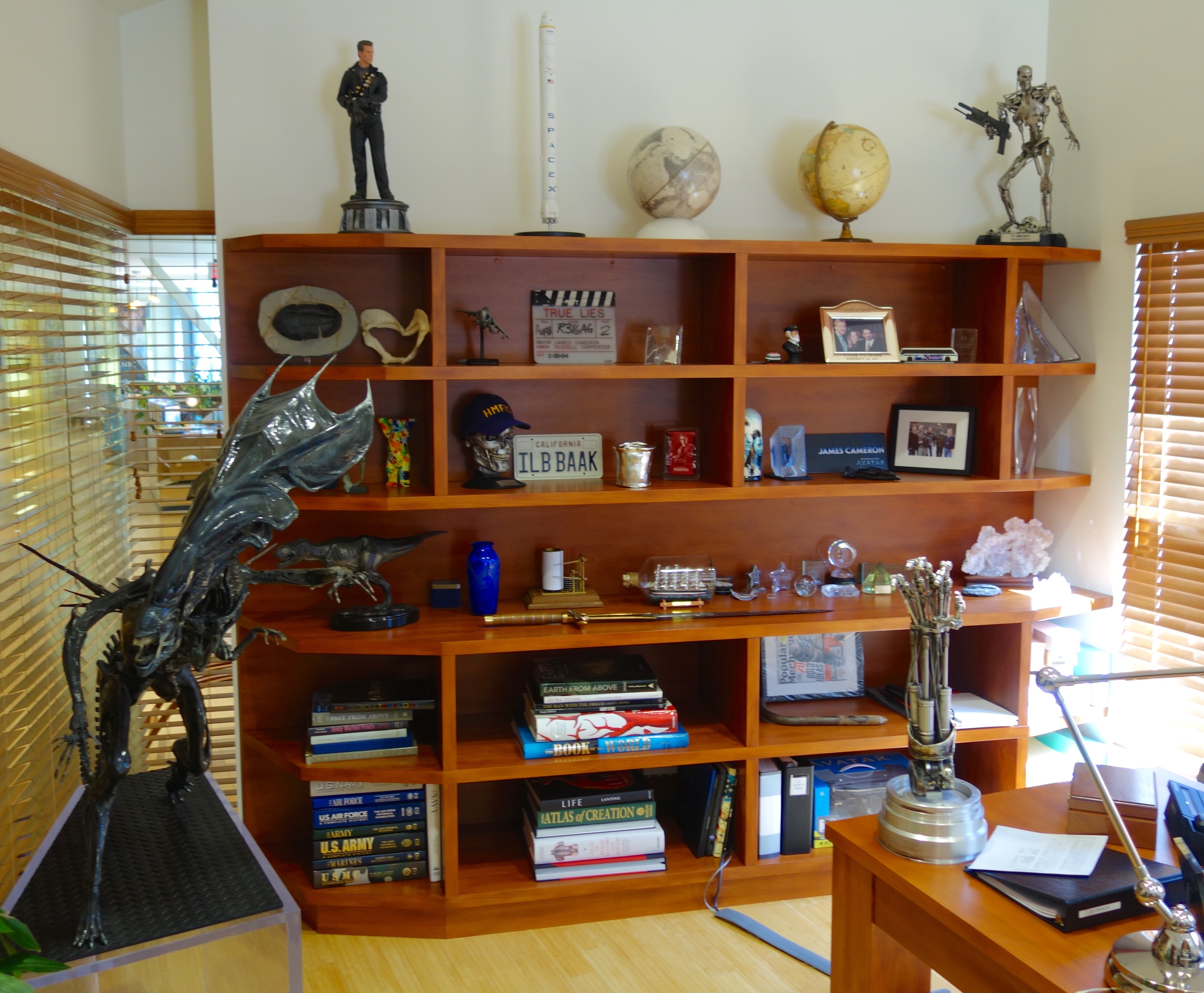The photograph depicts a detailed home office with an array of memorabilia and books carefully arranged on a prominent bookshelf set against a white painted wall. The highly organized shelf, which has rounded ends, is filled with a diverse collection of items including several books, frames with photographs, and glass statues or awards. Dominating the display are pieces that showcase a clear Arnold Schwarzenegger theme, including figurines of the actor as the Terminator, a hand from the Terminator movie, and a license plate that reads "I.L.B.B.A.A.K."—a nod to the iconic line "I'll be back." At the top of the shelf sits a globe, a white rocket, and another spherical object, while statues occupy both ends of the shelf. The scene also includes a large, peculiar gray statue with spiked edges resembling a fin or claw, possibly of an alien creature.

In the bottom right corner of the room, there is a light brown wooden desk adorned with a range of items: an adjustable silver-armed table lamp, a metal statue mounted on a base, a black binder topped with a white piece of paper, a brown wooden box, and the visible edge of a black keyboard. This office serves as a sanctuary for film memorabilia, especially from Arnold Schwarzenegger movies, creating a nostalgic and eclectic environment.